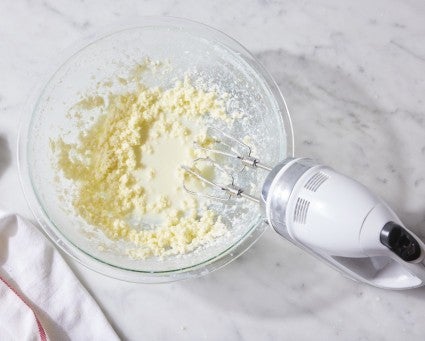This overhead photograph captures a pristine kitchen scene set on a white marble countertop with subtle gray streaks. At the center is a large, clear glass mixing bowl containing a clumpy, white mixture resembling whipped cream cheese. Resting on the side of the bowl is a white handheld electric mixer, its two wire beaters partially submerged in the mixture. The mixer features a black power button, adding a touch of contrast. A neatly folded white kitchen towel is visible in the bottom left corner of the frame, contributing to the meticulous arrangement of the setup. The scene exudes a sense of calm and readiness, indicating the initial stages of food preparation, potentially for a cream sauce or a dessert mixture.